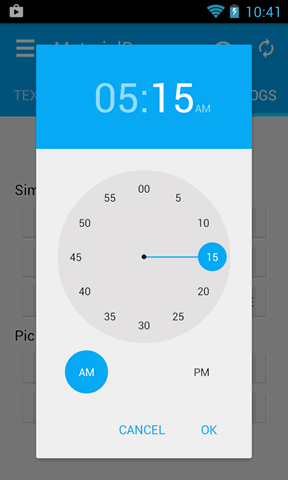In this detailed screenshot of a mobile device, the top left corner features the Google Play Store notification icon. In the top right corner, icons for Wi-Fi connectivity and battery level are present, along with a device time displaying 10:41. The central focus of the image is the alarm-setting page, specifically showing a clock interface where the user is configuring an alarm for 5:15 a.m. The interface prominently features a clock hand indicating the selected time. The background colors of the screen are predominantly black, blue, and white, creating a clear and visually distinct layout for setting the alarm.